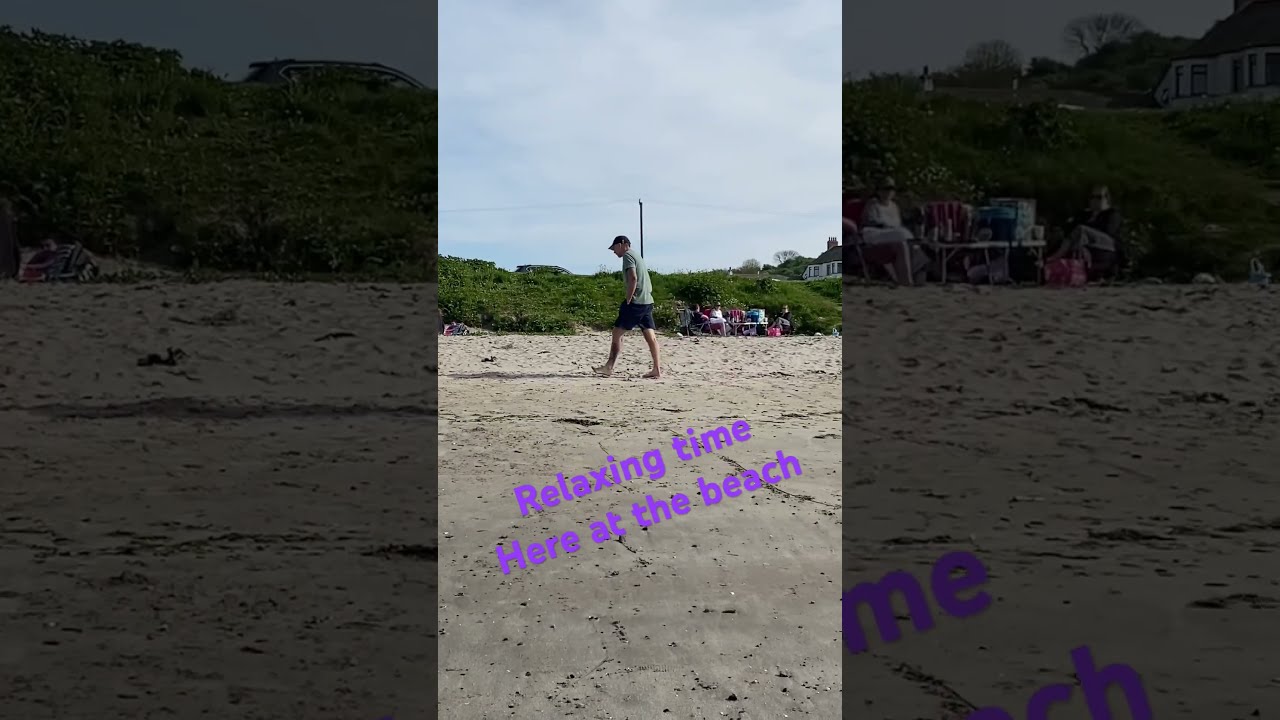A detailed image captures a serene moment at the beach. The central focus of the photo is a gentleman barefoot on the gray sand, wearing a green shirt, black shorts, and a dark baseball cap. He appears to be in his late 40s to 50s, looking downwards as he walks. Framing the main photo are two close-ups; the one on the left showcases the sandy shore and lush green grass with a car parked behind, while the right-side close-up features two people sitting on lounge chairs beside a picnic table, with camping gear and a house more clearly visible in the backdrop. The scene, possibly taken on a phone, is overlaid with bold, thick, purple text reading "relaxing time here at the beach," slanting diagonally from the bottom left to the top right. The setting suggests a peaceful, somewhat cloudy day, ideal for a family beach picnic against a backdrop of green bushes and a distant house perched on a small hill.